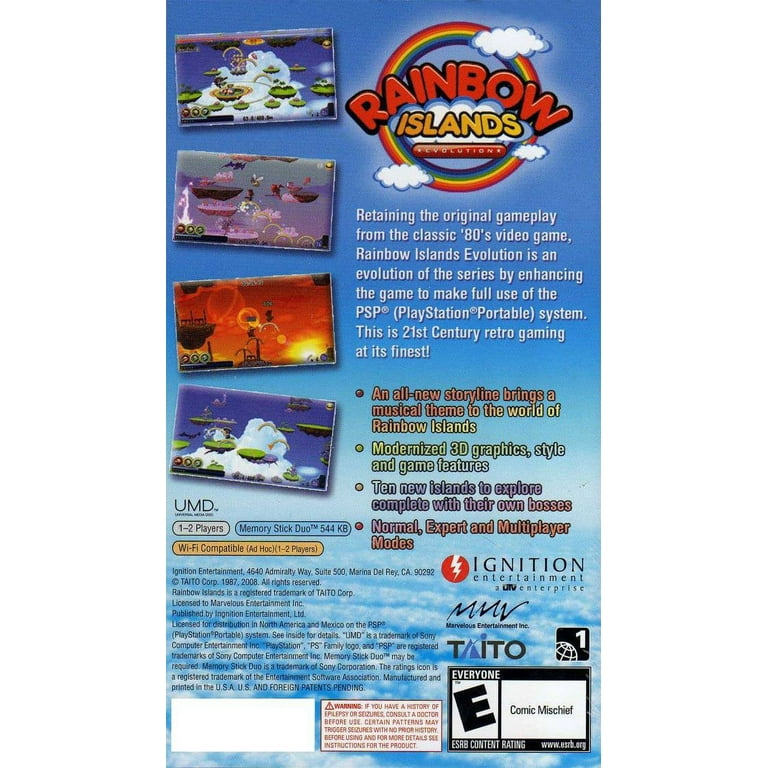The image appears to be the cover of a video game, "Rainbow Islands Evolution," designed in a horizontally aligned rectangular format. The background transitions from a solid blue sky at the top to light blue and white, indicating fluffy clouds towards the bottom. Dominating the upper right corner is a rainbow-colored circle featuring concentric arcs in red, yellow, green, blue, and possibly purple. Within this circle, "Rainbow" is written in red bubble letters, "Islands" in yellow bubble letters just below, and "Evolution" in white with stars flanking either side, all set against the sky and clouds.

To the left of the circle are four vertically aligned rectangular images, slightly tilted, showcasing screen grabs from the game. Below the game's title, a white paragraph reads: "Retaining the original gameplay from the classic 80s video game, Rainbow Islands Evolution is an evolution of the series by enhancing the game to make full use of the PSP (PlayStation Portable) system. This is 21st-century retro gaming at its finest."

Underneath this paragraph, there are four bullet points, each starting with text that shifts color. The bullets highlight: 
1. "An all-new storyline brings a musical theme to the world of Rainbow Islands" (orange).
2. "Modernized 3D graphics, style, and game features" (green).
3. "10 new islands to explore, complete with their own bosses" (purple).
4. "Normal, expert, and multiplayer modes" (dark orange).

In the lower right corner, a red circle with a lightning bolt inside indicates "Ignition Entertainment." Nearby, "Taito" is also noted. Lastly, there's a rectangular box rating the game as "E for Everyone" with a notation for comic mischief.